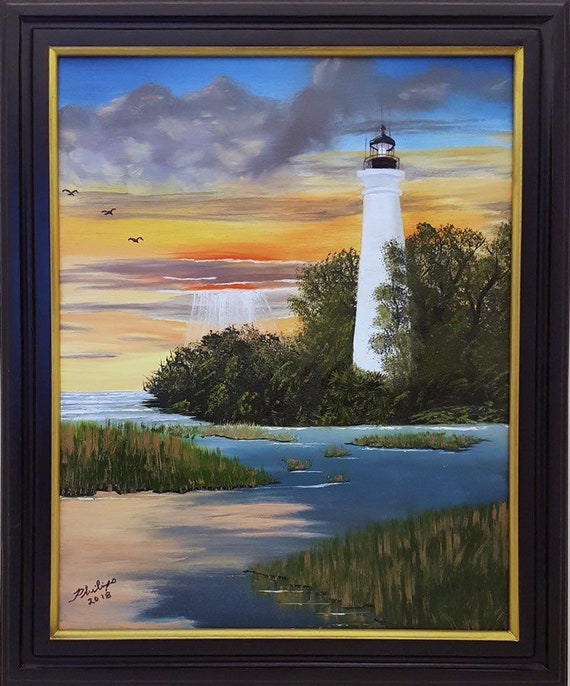The photograph captures a detailed view of a handmade piece of art housed in a dark blue or black frame with gold edging on the inside. The artwork, possibly created with pastels or oils, depicts a serene lighthouse scene at sunset. The top of the image showcases a blend of blue and purple clouds, gradually transitioning into a spectrum of yellows, reds, and oranges. Sunbeams break through the colorful sky, with a hint of red indicating the sun's presence.

In the top right corner, a white lighthouse with a black top is prominently featured, complete with a visible central light. The lighthouse is situated on marshland, surrounded by dense greenery and partially obscured by a tree. The foreground presents a blue body of water reflecting the sky above, interspersed with patches of grass and terrain, including brown sand fading into the water from the left.

Further details include three birds flying in the distance on the left side and the artist's signature, "Phillips 2018," handwritten on the bottom left of the painting. The composition skillfully blends colors, creating a harmonious and vibrant sunset scene.